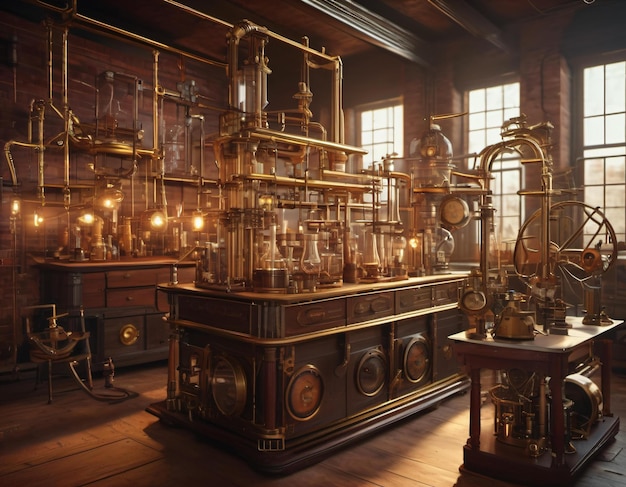The image depicts a vintage, turn-of-the-century laboratory inside an old-fashioned building. It's a computer-generated or graphic image that remarkably mimics a photograph. The setting features three large lab tables arranged in a three-quarter view. The front table is smaller, followed by a longer table, and a taller table in the background. Each table is cluttered with an assortment of equipment, including glass beakers, various oddments, and some unique contraptions reminiscent of large wheels or turbines. An elaborate system of copper pipes runs both horizontally and vertically throughout the room, descending from the ceiling and connecting to the tables. Some of these pipes lead to circular doors and small cabinet-like structures beneath the tables, bearing a resemblance to washing machines seen in laundromats.

The room is dimly lit by a combination of candlelight and a few lit lanterns scattered among many unlit ones, adding to the antique atmosphere. The backdrop includes walls with additional equipment or piping, with wooden rafters overhead similar to those found in old New York buildings. The light filtering through three large windows at the back bathes the wooden floor, creating reflective patterns, and subtly illuminating the scene. There's a hint of an urban landscape visible through the windows, further grounding the lab in an old, industrial-era setting.